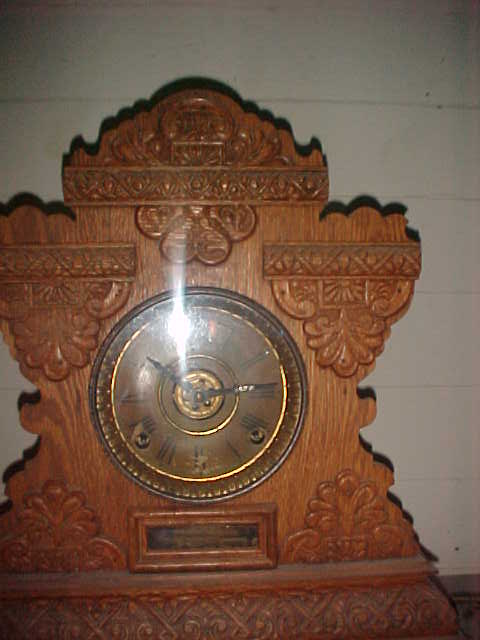This image features an elegant, antique wooden clock reminiscent of a grandfather clock. The clock exudes a sense of timelessness and history, highlighted by its intricate craftwork. The wood is adorned with delicate, Bohemian-style floral patterns, intricately carved into the surface at the bottom and sides, creating a sophisticated embroidery-like effect. 

At the center of the clock is a large, golden-plated frame housing the clock face, which prominently displays black Roman numerals and matching black clock hands, adding a classic touch. Just above the base, there is a rectangular carved-out section whose purpose remains unclear, adding a hint of mystery to the elaborate design.